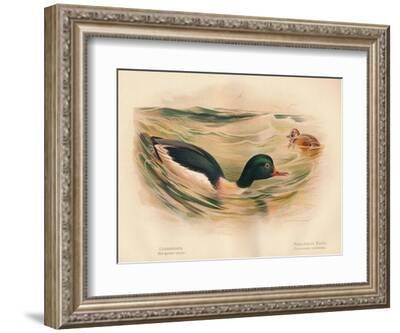This photograph features a framed painting or print depicting a serene nature scene. The artwork is presented on off-white paper, matted with a pristine white matte, and encased in an ornate silver-colored frame. The frame is positioned upright, tilted slightly to provide a three-dimensional perspective against a minimalist white background. The primary subject of the painting is a duck with a striking metallic black and green head and back, as well as a white neck and underside of its wing. The duck has a distinct yellow eye and a red beak, and it is oriented to the right. This duck is partially submerged, with its lower body hidden by the water it floats in. Close behind this main duck, positioned slightly up and to the right, is a smaller duck with a mottled brown appearance. Both ducks swim in a lustrous circular swirl of golden, green, and gray hues, representing the water. The overall composition elegantly captures the tranquil beauty of these ducks in their aquatic environment.